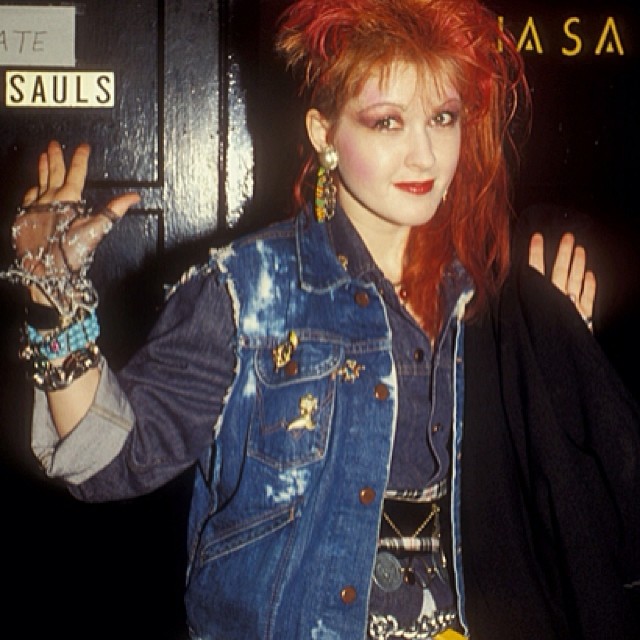The detailed color photograph showcases Cindy Whopper standing in front of a black door and wall, partially obscuring yellow letters that read "ASA" and the name "S.A.U.L.S." Cindy is smiling without showing her teeth, with her arms raised at her sides. She is attired in a sleeve-cut denim vest, adorned with gold buttons, pins, and a silver chain hanging from it. Under the vest, she wears a long-sleeved, button-up denim shirt with black buttons, its sleeves rolled up just below her elbows. Her ensemble is complemented by beaded bracelets and sheer, fingerless gloves on her wrists. She carries a black garment in one arm. Cindy's striking hairstyle features long red hair on one side and an almost-shaved look on the opposite side. Heavy red lipstick and purple eyeliner accentuate her makeup. Large metal circular earrings with multicolored dangling parts complete her bold look.